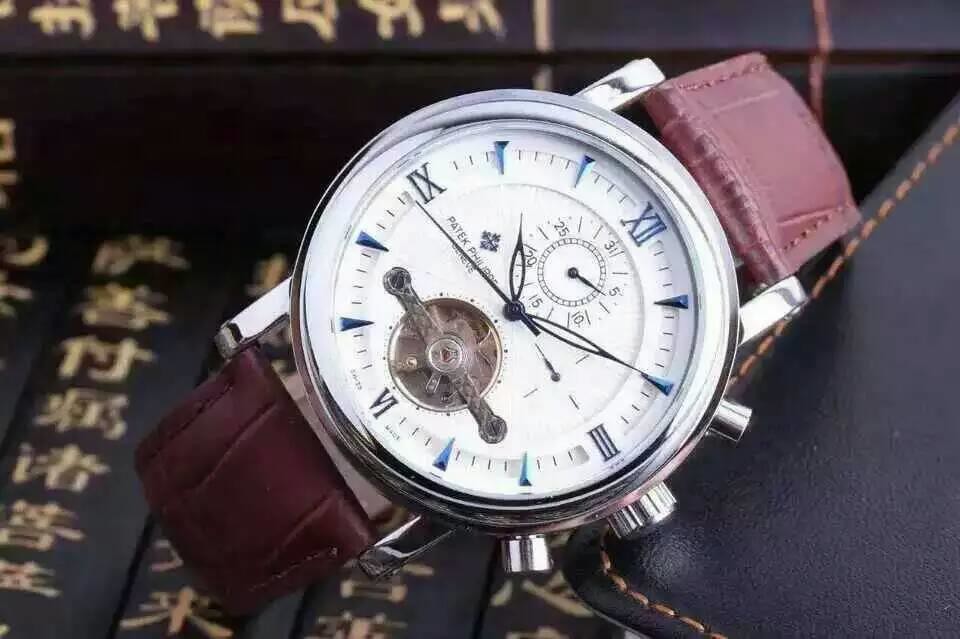In the foreground, a meticulously crafted wristwatch draws immediate attention with its sophisticated design. The watch features a classic silver case and a detailed silver dial that displays the hour hand poised between 10 and 11, the minute hand at 2, and the second hand slightly before 9. The watch is complemented by rich brown leather straps, elegantly stitched along the edges, and secured to the case with sturdy metal lugs. On the right side of the watch face, a collection of small cylinders and a detailed dial add to the intricacy of the timepiece, while various dashboard-like markings are evident around the circumference of the dial.

In the top left corner, Chinese characters provide a hint of cultural richness, contrasting with the mechanical precision of the watch. The bottom left of the image is filled with neatly arranged rows of books, each bound in a way that showcases an array of Chinese characters on their spines. Finally, the rightmost edge of the image features a piece of black leather with decorative stitching, perfectly balancing the composition and adding a touch of textural contrast. This image uniquely melds elements of Eastern literature and Western horological craftsmanship, creating a harmonious blend of tradition and technology.